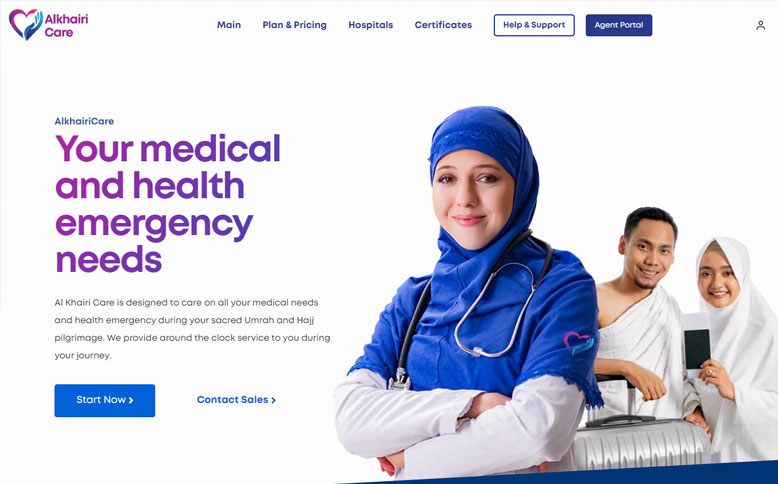The ALKHAIRI website's interface features a distinct layout. Positioned on the upper left corner is the ALKHAIRI logo, with the word "CARE" beneath it in a smaller, purple font. Adjacent to this logo is an icon of a heart. Extending to the right and center-aligned is a horizontal navigation menu with options in blue font, reading: "MAIN," "Plan and Pricing," "Hospitals," and "Certificates." Further to the right, the "Help and Support" button is prominently displayed, alongside the "Agent Portal" link.

Below this top section, the main area of the website is divided into two sections. On the left, bold purple text states, "Your Medical and Health Emergency Needs," followed by a four-line paragraph in a smaller black font elaborating on the offerings. Underneath this text, there is a prominent blue "Start Now" button. Positioned to its right is a "Contact Sales" hyperlink, also in blue font. The right side of this central section features an accompanying image that complements the textual information on the left.